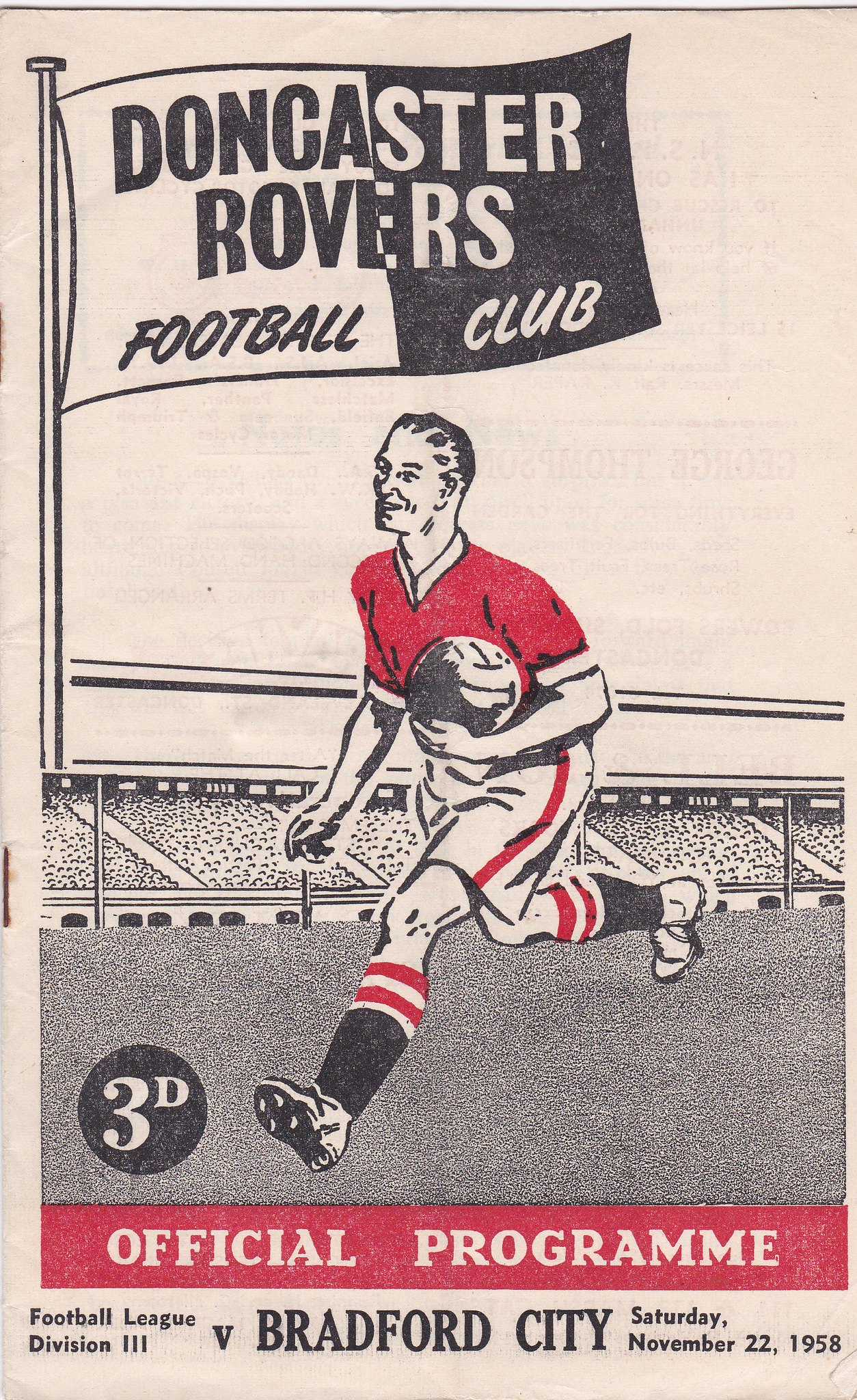The image depicts a vintage football club program for Doncaster Rovers, colored in white, gray, black, and red. At the top of the program, there is a cartoonish, hand-drawn flag on a flagpole, with the left half of the flag in white featuring black text, and the right half in black with white text, reading "Doncaster Rovers Football Club." The sky in the background is white. Below the flag, a hand-drawn figure of a man wearing a red T-shirt, white shorts with red stripes, and black socks with white and red stripes on the calves is running with a soccer ball in his hand. He is depicted in an action pose, as if crossing a field, with an abstract, indistinct crowd in the stadium stands behind him. Toward the bottom of the program, a bold red stripe features white text that reads "Official Program." Below this, against a white background with black text, is written "Football League, Division III, Bradford City," followed by the date, "Saturday, November 22, 1958."